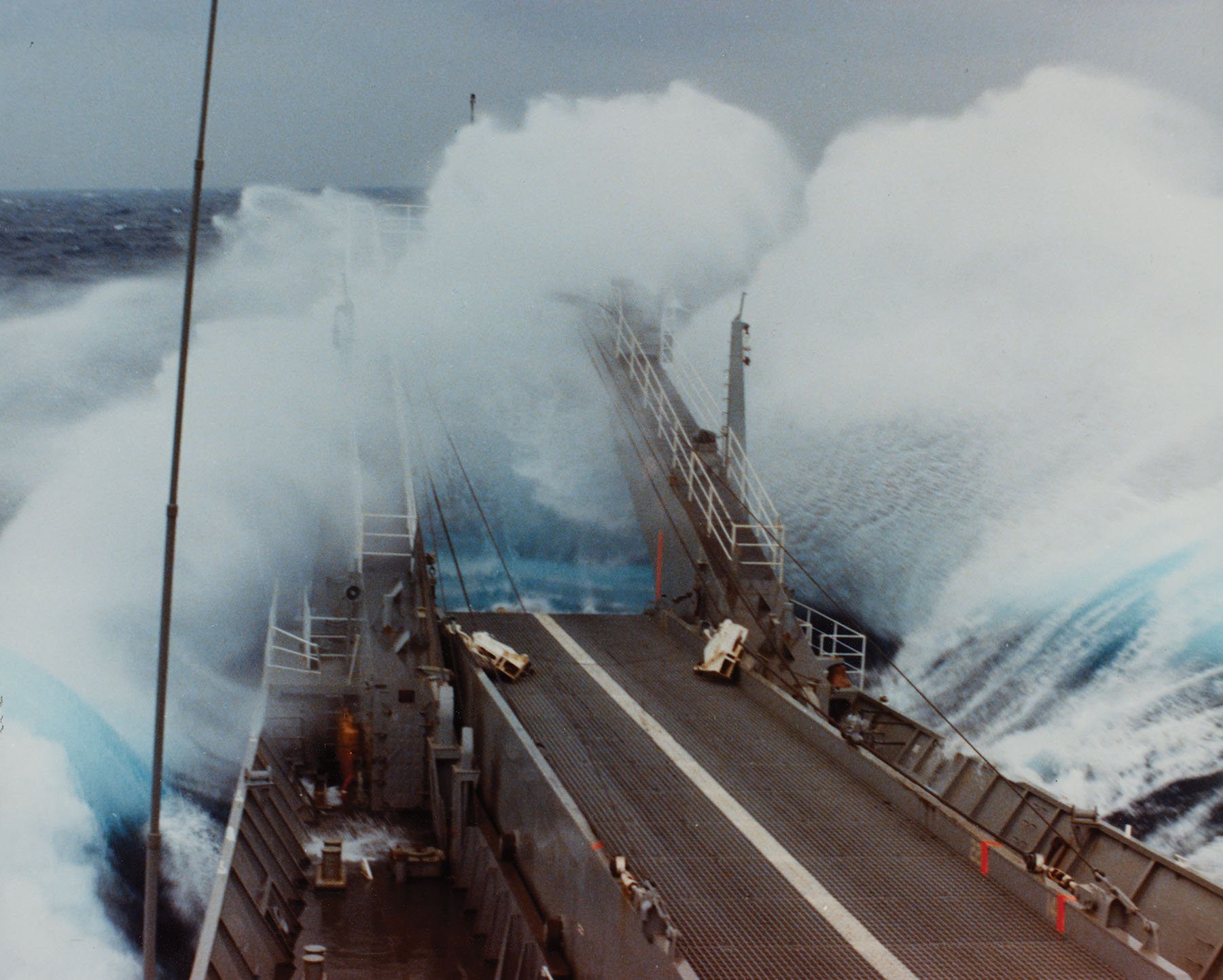The image depicts the deck of a large ship navigating through a tumultuous sea. The metal surface of the deck is laden with wooden pallets scattered across various spots. Several cranes extend from the back of the ship, with one crane particularly notable, where a man stands nearby. The vessel is battling rough seas, with massive waves surging above and splashing onto the deck, creating a mixture of mist and white foam. The ocean's color shifts from dark blue in the background to a lighter cyan near the ship. The deck is marked by a solid white line running down its center, and red paint indicating certain areas. Rusted materials, resembling pallets, lie around the deck. The surrounding sky is filled with dark, gray clouds, allowing only limited natural light to seep through, adding to the overall dramatic and foreboding atmosphere. White railings line the sides of the ship, contrasting with its dark, possibly brown, and worn appearance.